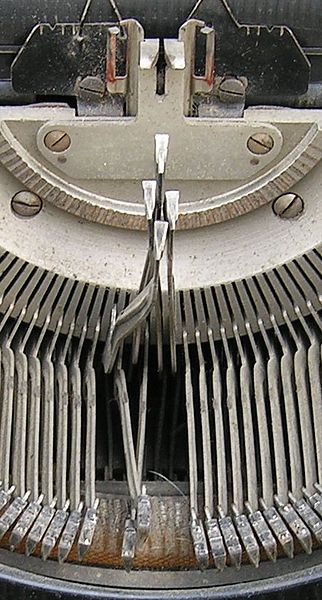A close-up photograph of a piece of machinery, possibly an automotive component, showcases its intricate details and current state of disrepair. The focal point features numerous metal appendages, primarily oriented downward, with a few conspicuously out of place, jutting upwards, possibly indicating missing or broken parts. Above these appendages, a series of U-shaped brackets securely fasten the structure together, while at the top, distinct black components resembling cat ears add a peculiar visual contrast. Additional screws at the apex, bearing more wear and a different coloration, suggest extensive use. The entirety of the machinery is coated in a light tan hue, with visible rust accumulating at the lower section, underscoring its aged and possibly incomplete or malfunctioning condition.